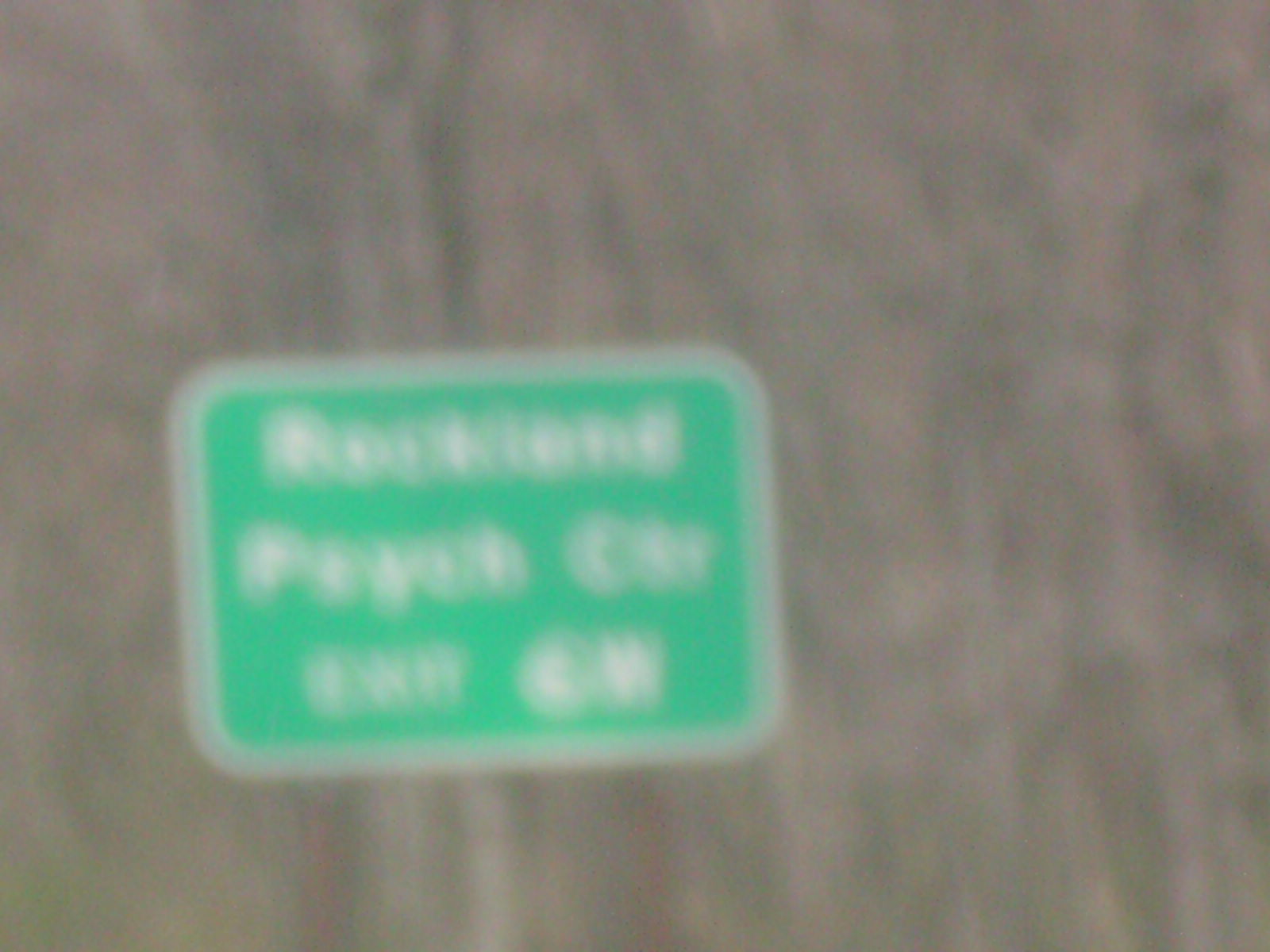A blurred image captures a green road sign with a white border and indistinct white lettering. The text on the sign is difficult to decipher due to the focus issue, but the first word appears to start with an 'R', the second with a 'P', and a shorter third word possibly starts with a 'C'. The final word seems to repeat the third word, though this is also uncertain. The surrounding environment is predominantly brown and fuzzy, making it hard to distinguish specific details outside of the sign itself.